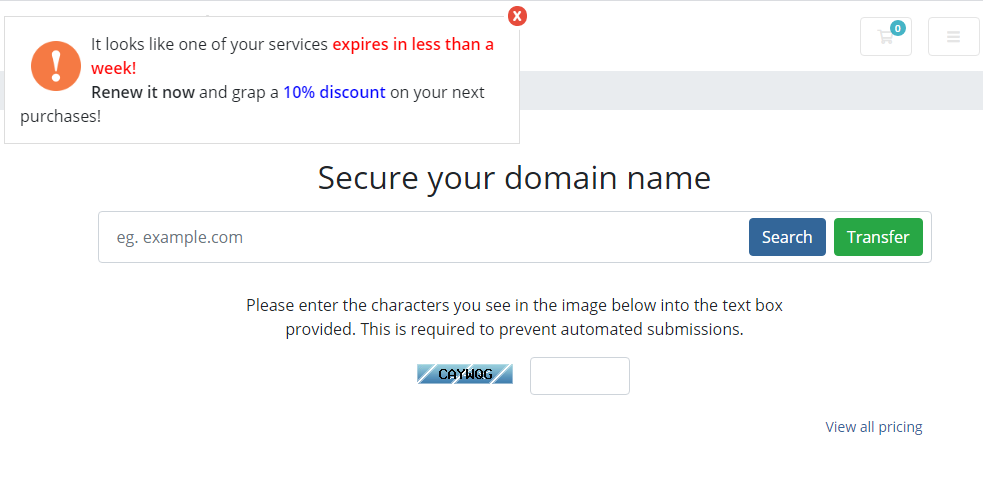This is a screenshot of a specific section of a website. The background is predominantly white. 

In the upper left corner of the image, there is a prominent pop-up window framed by a white rectangle, which features a red circle with a white 'X' in the upper right corner for closing the pop-up. Inside the pop-up is a notification in black font that reads: "It looks like one of your services expires in less than a week," with the phrase "less than a week" highlighted in red font. To the left of this text, there is a red circle with a large white exclamation mark inside it.

The pop-up continues to provide a call to action beneath the initial notification: "Renew it now and grab [sic] a 10% discount on your next purchases," displaying a typographical error where "grab" is incorrectly spelled as "G-R-A-P". This section is overlaid on a gray bar for emphasis.

In the upper right section of the screen, outside of the pop-up, there is a shopping cart icon indicating access to the user's cart.

Below the gray bar, the website offers an input area captioned with "Secure your domain name," including a text field prompting users to enter a domain name example, such as "eg.example.com." To the right of this field, there are two buttons: a purple button labeled "Search," and a green button labeled "Transfer."

Further down, there is a CAPTCHA verification section. It prompts users with the text: "Please enter the characters you see in the images below into the text box provided. This is required to prevent automated submissions." Beneath this instruction, there is a blank input field followed by a CAPTCHA challenge displaying the characters "KWAG."